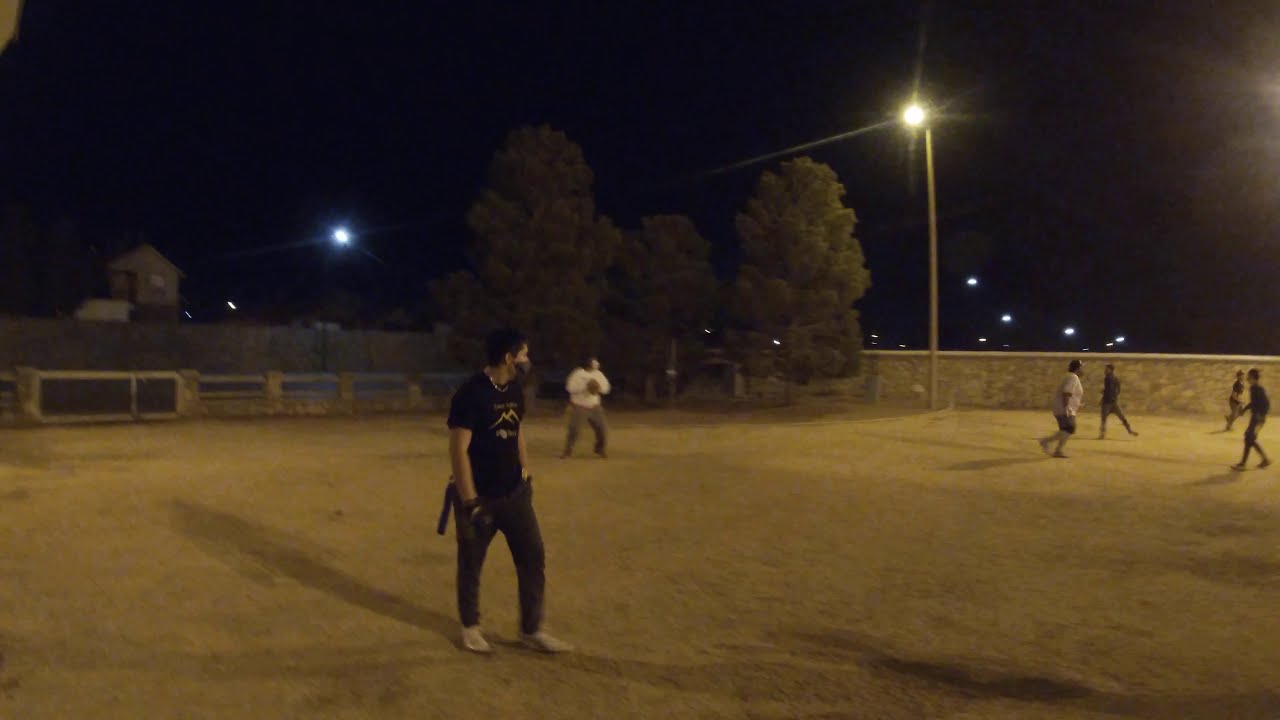In the photograph taken at night, six individuals stand in an expansive, flat lot illuminated by a large streetlight. The background reveals a fence with horizontal cement bars and, to the right, a brick wall. The ground appears sandy and there are several focused streetlights and a tiny shack visible in the distance. The person closest to the camera, positioned toward the left, is clad entirely in black, including a shirt, face mask, pants, gloves, and white shoes. Behind him, another individual wears a white shirt and gray pants, holding a football, seemingly ready to pass it. To the right, four more individuals stand, three dressed in black and one in white, appearing as though they are waiting for the play. The scene suggests a group of friends playing a casual night game, possibly football, in this enclosed lot. Several trees line the perimeter, adding to the ambiance of a late-night outing under the streetlights.